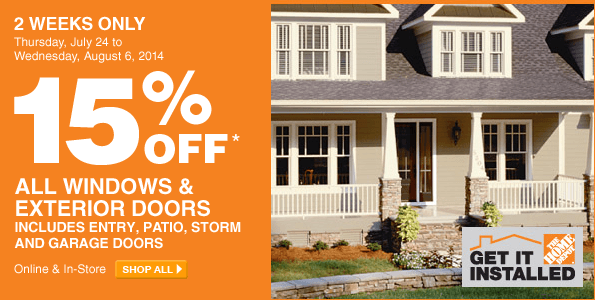In this image, you see a charming house set in the background, featuring multiple windows and a prominently displayed door. A staircase with several steps leads up to a welcoming veranda adorned with various plants and greenery. To the left of the image, a promotional banner from The Home Depot is visible, announcing a special offer that lasts for two weeks only, from Thursday, July 24th, to Wednesday, August 6th, 2014. The banner highlights a 15% discount on all windows and exterior doors, including entry, patio, storm, and garage doors. The offer applies to items purchased online or in-store, with an option for installation services.